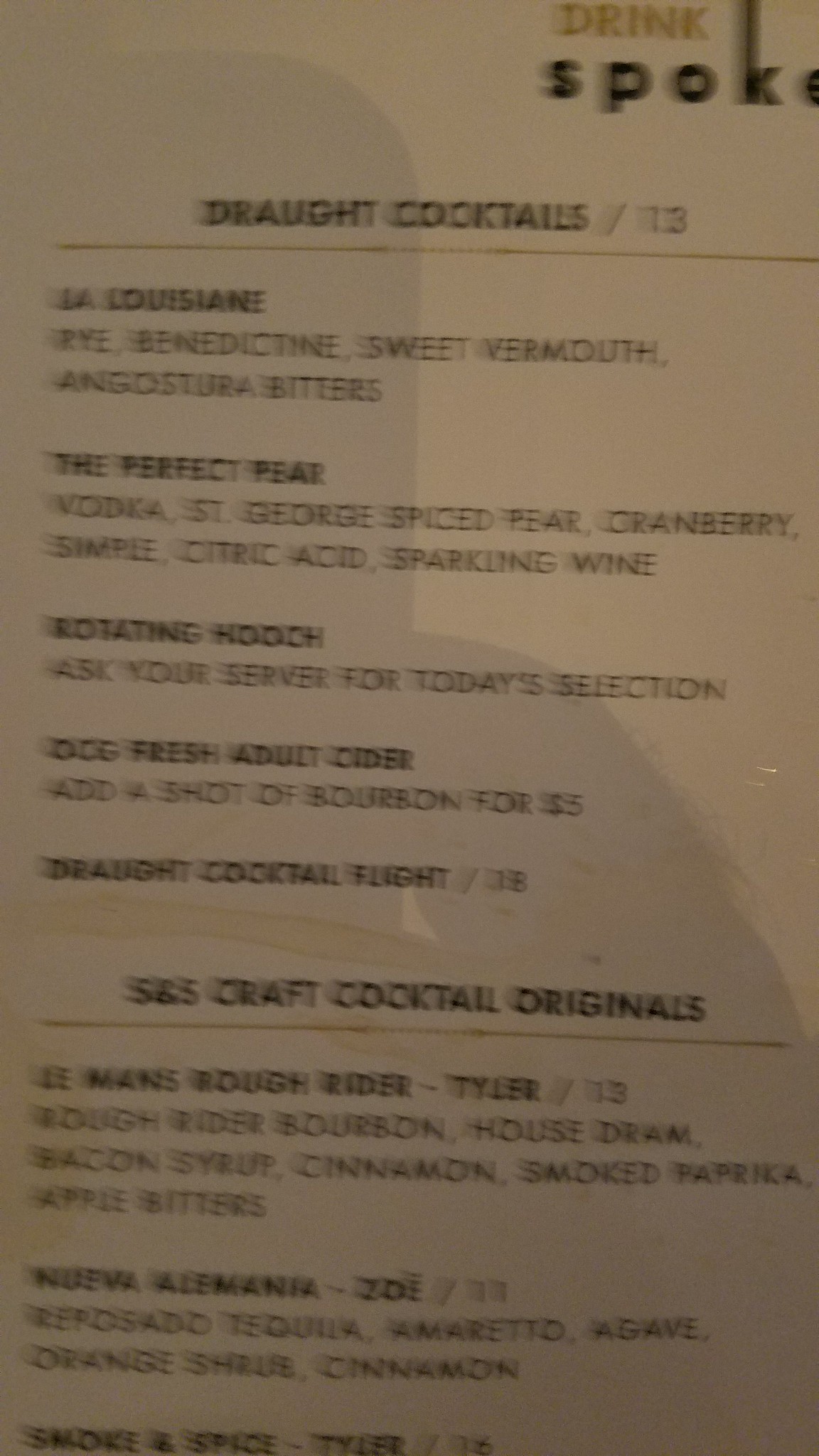This is a rather blurry photograph, vertically framed, clearly taken with a phone. It captures part of a draft cocktails menu from a bar or restaurant. At the very top, partially obscured, it reads "Drink Spoke," possibly indicating "Drinks Spokane" or a similarly named bar. The menu details draft cocktails priced at $13 each. The shadow of a hand holding the phone is visible in the image, adding to its lack of clarity.

The menu features several enticing cocktail options:

1. **La Louisiane** - Comprising rye, benedictine, sweet vermouth, and angostura bitters.
2. **The Perfect Pear** - Made with vodka, St. George's Spiced Pear, cranberry, citric acid, and sparkling wine.
3. **Rotating Hooch** - Encouraging patrons to ask the server for today's special selection.
4. **OCG Fresh Adult Cider** - Option to add a shot of bourbon for $5.
5. **Draft Cocktail Flight** - Priced at $18.

Further down, another section highlights "5&5 Craft Cocktail Originals":

- **LaMont's Rough Rider-Tyler** - Features Rough Rider bourbon, house gram, bacon syrup, cinnamon, smoked paprika, and apple bitters, for $13.
- **Nueva Armenia-Zoe** - Priced at $11, it includes tequila, amaretto, agave, orange shrub, and cinnamon.
- A partially obscured cocktail named **Smoke and Spice-Tyler** - Costs $16, but details of its ingredients are cut off in the photograph.

The menu is set against a white or off-white background, with faint reflections and shadows indicating it might be behind glass.